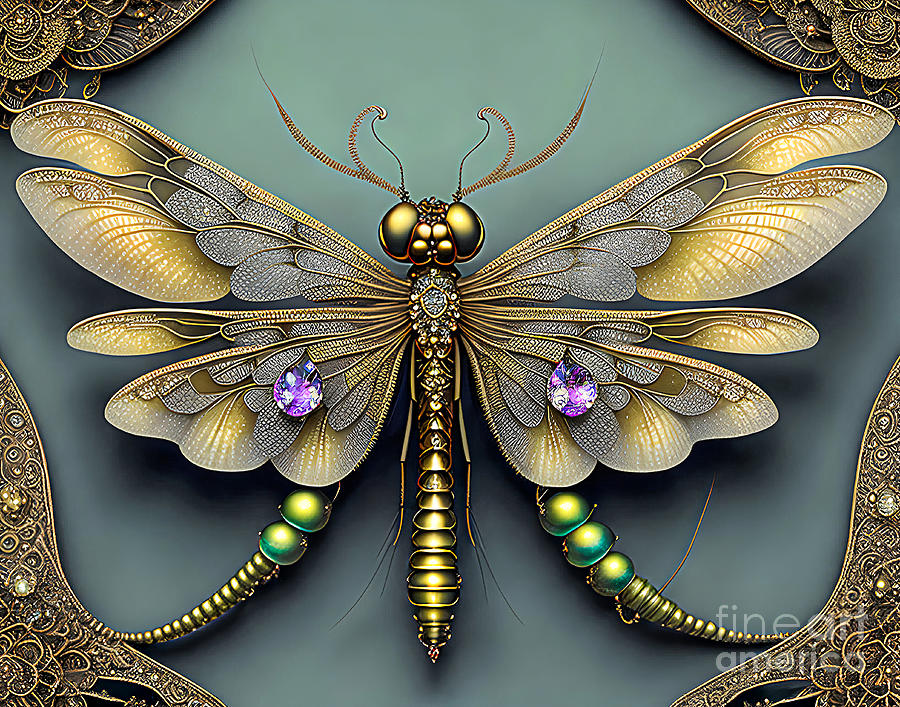The image portrays a highly detailed piece of artwork or jewelry, most likely a pin or ornament, depicting a butterfly. The butterfly is crafted in gold with intricate designs, featuring a blend of precious stones. The body of the butterfly is adorned with diamond-like stones, while the wings exhibit purple stones. The leg areas beneath the wings have green accents, and additional details include white and blue diamond-like drops on the back wings. Extending from the back of the butterfly are small, globe-like structures and diminishing cylindrical forms. Surrounding the butterfly, there is a border on both sides and top, with elaborate patterns in gold and silver, all set against a bluish-gray background. The piece strikes a balance between detailed craftsmanship and rich color use, combining elements that suggest both physical jewelry and digital artwork.